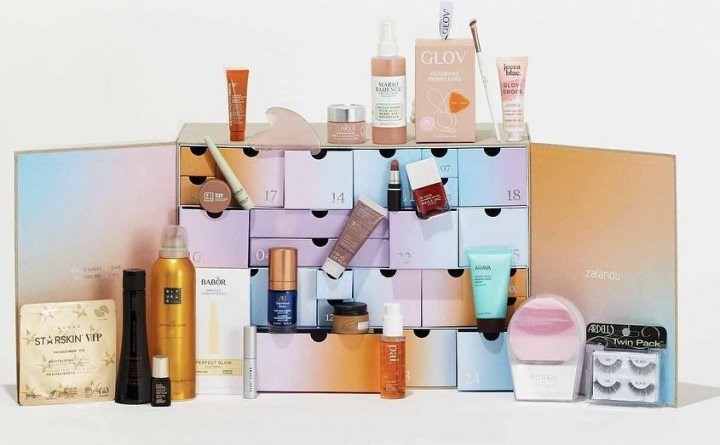This photograph depicts an intricately designed storage box, likely made of cardboard and covered in fabric. The box features numerous drawers of varying sizes, each adorned with a number, including 14, 17, 18, 22, and 25. The drawers are painted in pastel colors, adding a charming aesthetic to the overall design. The drawers have semi-circle cutouts at the top, serving as convenient finger pulls for easy access.

On the bottom row, a particularly wide drawer stands out, while a few other wide drawers are positioned halfway up. In the top left corner, several tiny drawers are visible, contributing to the assortment of drawer sizes. The box is open, with its side panels flared out, revealing an orange and blue painted right panel that prominently displays the word "Z-E-F-A-N-D-O."

In front of the box, a variety of beauty products are scattered, including a twin pack of fake eyelashes, a rounded container with a pink lid filled with a white substance, and a small spray bottle. Additionally, there are various squeeze and spray bottles dispersed across the scene, enhancing the organized yet bustling atmosphere of this storage setup.